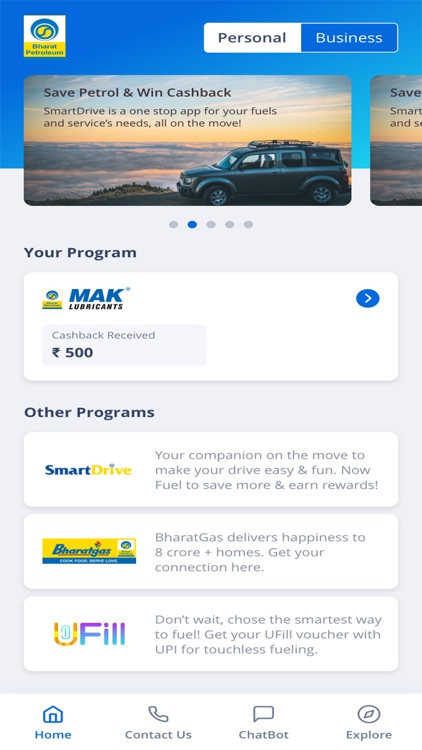In this screenshot, we see a webpage with a blue header at the top. In the upper left corner of the header, there is an unclear logo featuring a square design with a white box on top and a round circle icon with a yellow bottom inside it. The word "Petroleum" is partially visible within the logo. To the right of the logo, there are two buttons: a white button labeled "Personal" and a blue button labeled "Business."

Beneath the header, there is a colorful photograph of a Jeep-like vehicle parked alongside the ocean, with its nose pointing west. The vehicle has a roof rack carrying what appears to be a surfboard, and the sky in the background is painted with sunset hues. Overlaying this image is dark blue text that reads, "Save petrol and win cash back. Smart Drive is a one-stop app for your fuels and services needs. All on the move."

Below this image, in a white box, we see bold blue text that reads "Mac" and beneath that, the word "Lubricants" is displayed. Further down in a light blue section within the white box, it mentions "Cash back received 500."